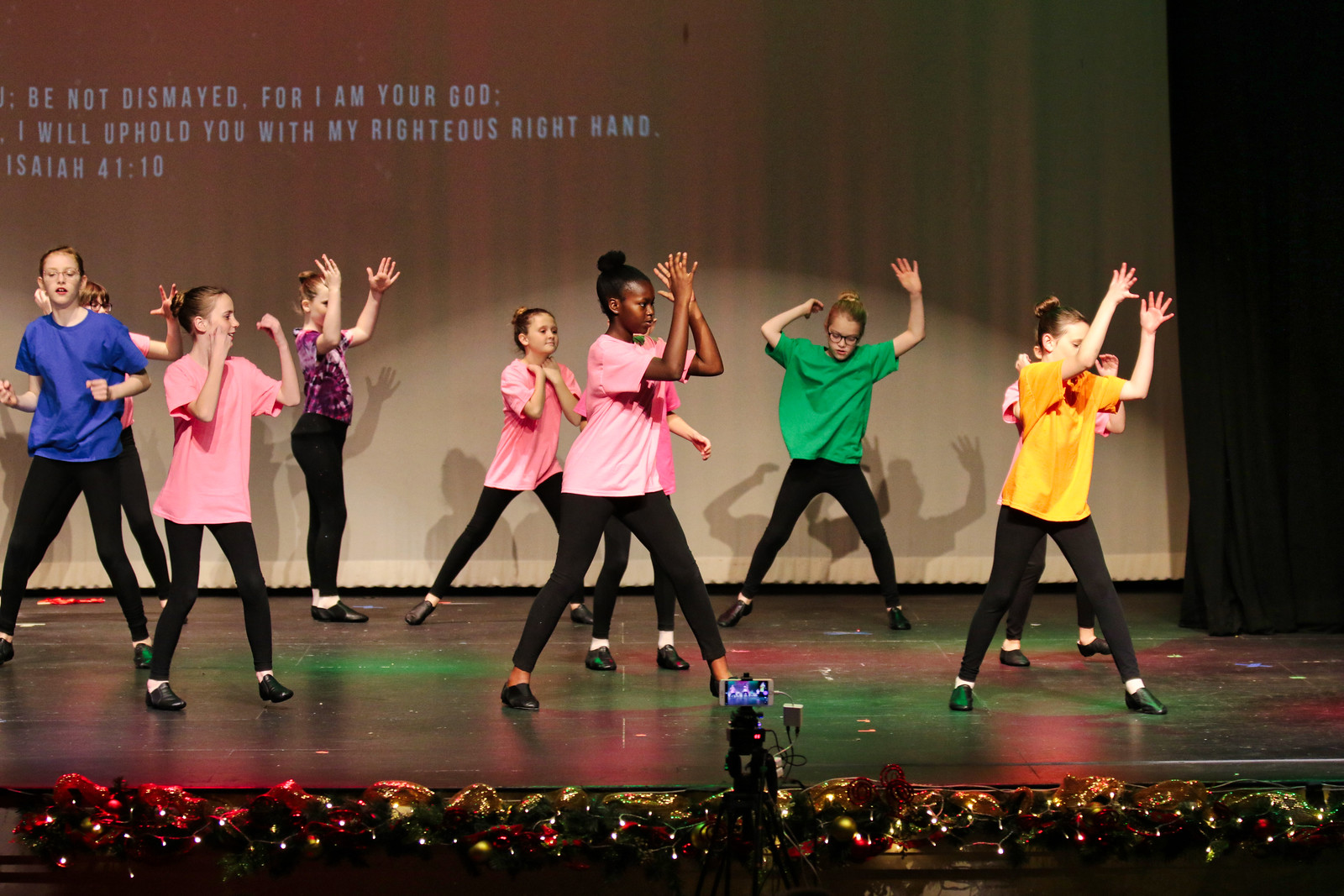The image captures a lively school play or church performance featuring a group of young girls on a stage adorned with festive holiday lights and decorated with flowers and wreaths. The children, appearing to be of different races, are dressed in black tights and shoes, each sporting a different colored t-shirt—pink, blue, green, yellow, and even purple. They are energetically dancing with their hands raised in the air, facing mostly towards the right side of the frame. In the background, a white curtain displays an inspiring Bible verse, "Be not dismayed, for I am your God. I will uphold you with my righteous right hand" from Isaiah 41:10. The scene is captured from what seems to be the front row, and a phone on a tripod set up near the front of the stage records the joyful performance.